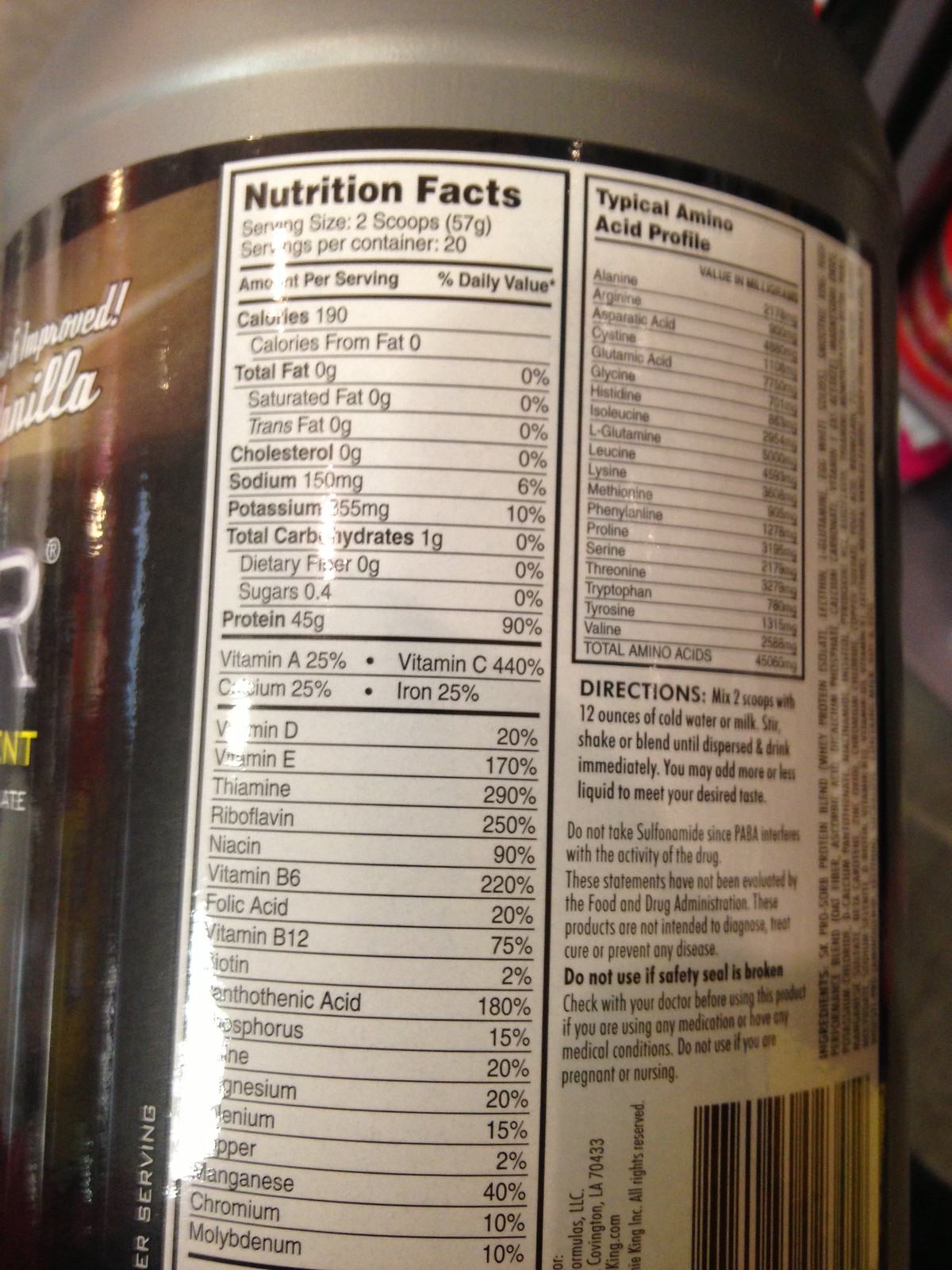**Product Caption: Detailed Nutrition Facts for Protein Shake**

The image showcases the back label of a protein shake bottle, focusing on the detailed Nutrition Facts. The label specifies the serving size as 2 scoops (57 grams), with a total of 20 servings per container. Here is a breakdown of the nutritional information per serving, along with their daily percentage values:

- **Calories:** 190 
- **Calories from Fat:** 0
- **Total Fat:** 0 grams 
- **Saturated Fat:** 0 grams
- **Trans Fat:** 0 grams
- **Cholesterol:** 0 grams
- **Sodium:** 150 mg (6%)
- **Total Carbohydrates:** 1 gram (0%)
- **Dietary Fiber:** 0 grams (0%)
- **Sugars:** 0.4 grams (0%)
- **Protein:** 45 grams (90%)

The label also lists a range of vitamins and minerals including:

- **Vitamin A:** 25%
- **Vitamin C:** 440%
- **Calcium:** 25%
- **Iron:** 25%
- **Vitamin E:** 20%
- **Vitamin E:** 170%
- **Thiamine:** 290%
- **Riboflavin:** 250%
- **Niacin:** 90%
- **Vitamin B6:** 220%
- **Folic Acid:** 20%
- **Vitamin B12:** 75%
- **Biotin:** 2%
- **Pantothenic Acid:** 180%
- **Phosphorus:** 15%
- **Magnesium:** 20%
- **Selenium:** 20%
- **Copper:** 22%
- **Manganese:** 40%
- **Chromium:** 10%
- **Molybdenum:** 10%

There is also a typical amino acid profile displayed on the label, although it is not fully legible in the image.

**Directions:** Mix two scoops with 12 ounces of cold water or milk. Stir, shake, or blend and drink immediately. Adjust the amount of liquid to achieve your desired taste.

**Warnings:**
- Do not take with sulfonamide as it may interfere with drug sensitivity.
- The product is not intended to diagnose, treat, or cure any disease.
- Do not use if the safety seal is broken.
- Consult a doctor before using this product if you are on medication or have any medical conditions.
- Do not use if you are pregnant or nursing.